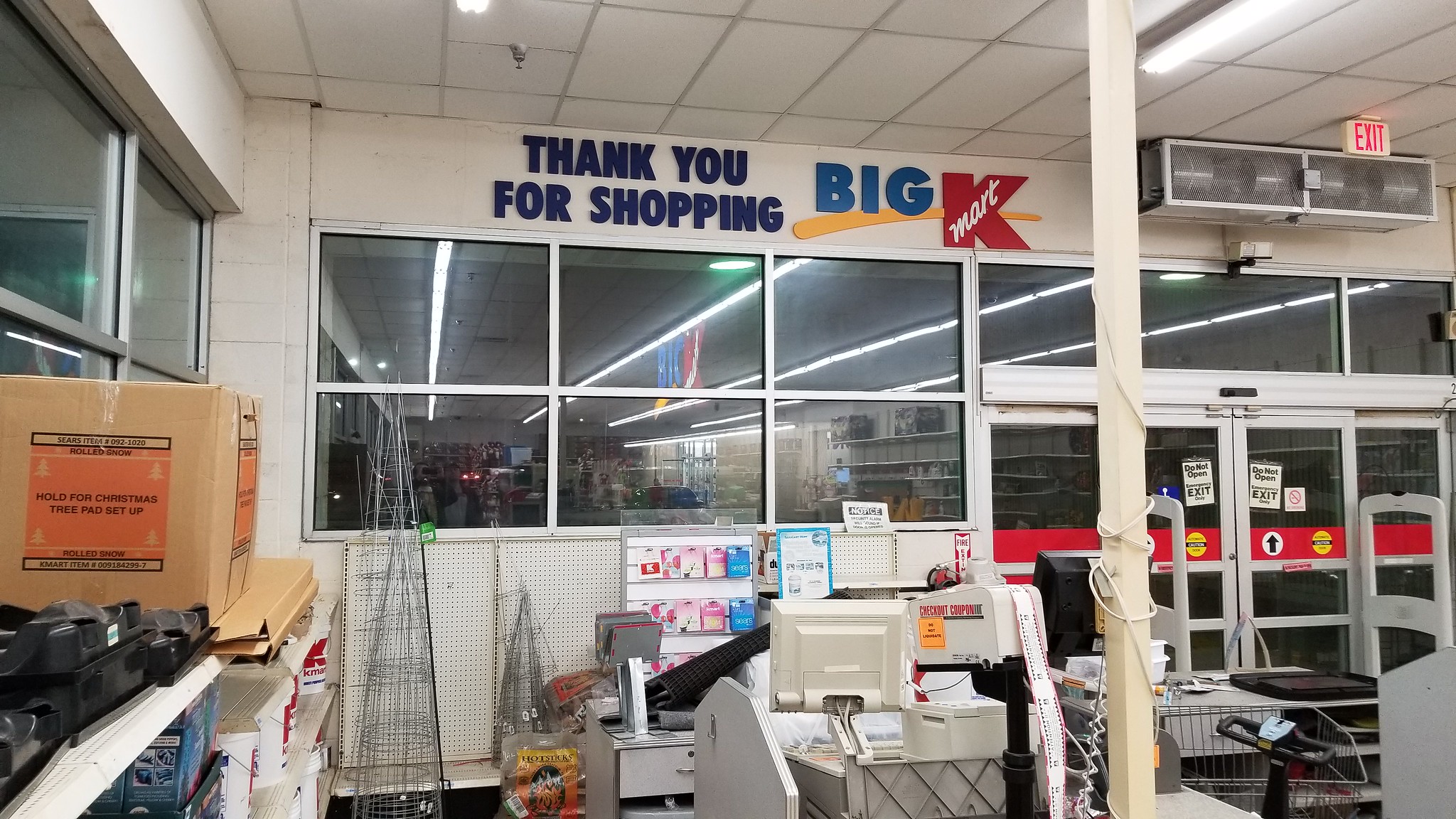A bustling entrance to Big Kmart greets visitors with a blend of functionality and a warm farewell. In the foreground on the right, a checkout lane invites customers to complete their purchases, while on the left, shelves neatly lined with colorful buckets catch the eye. The automatic sliding doors, marked with a yellow caution sign, usher shoppers in and out effortlessly. Above the entrance, just below the ceiling, a prominent sign expresses gratitude with the words, "Thank you for shopping." The entire scene encapsulates the welcoming and organized atmosphere of the department store.